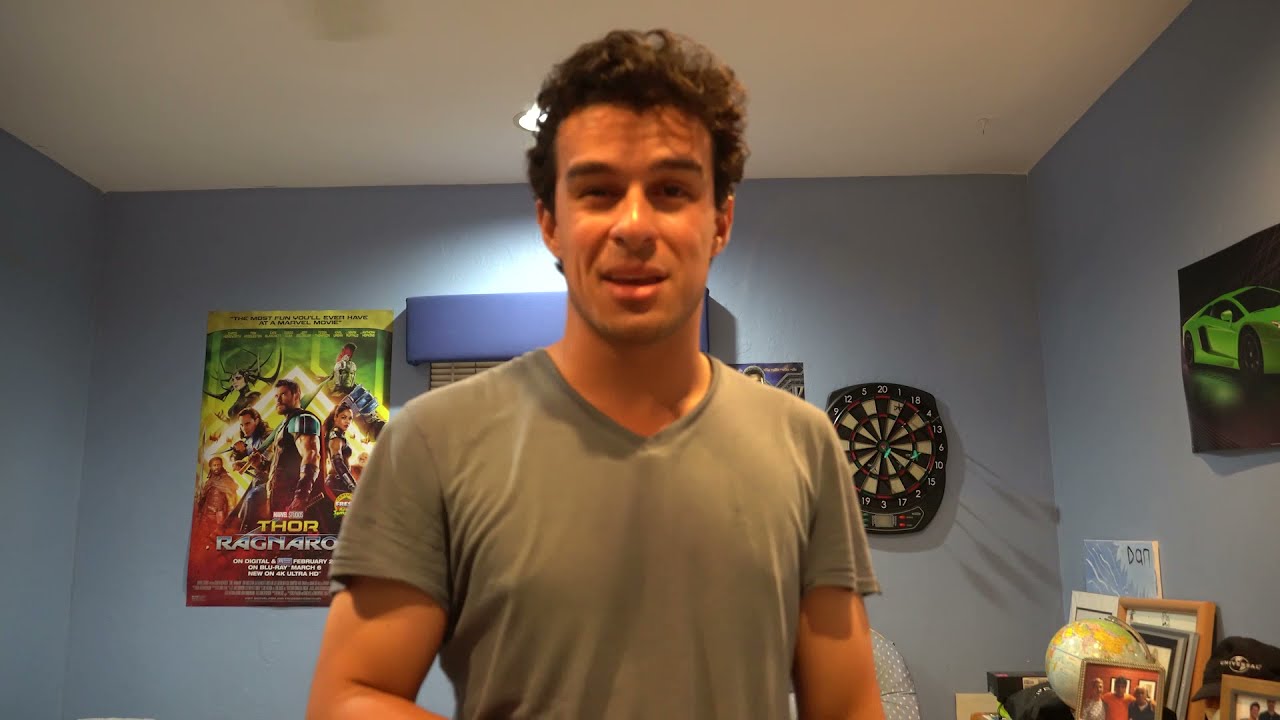The image depicts a room with blue walls and a white ceiling, decorated with various items suggesting a young boy’s bedroom. Central in the image stands a man, likely in his 20s or 30s, with short, styled brown curly hair. He appears to be talking, his front teeth visible, while wearing a green V-neck short-sleeved t-shirt. Directly behind him is a window with white blinds, topped with a blue valance. To his left, on the blue wall, hangs a "Thor: Ragnarok" movie poster. On his right, there's a black dartboard and a desk cluttered with framed pictures and a small globe. Additionally, on the right wall, there is a poster of a green sports car. The room also contains hints of other colors such as gray, green, yellow, brown, orange, red, peach, black, and white, detailing various elements throughout the space.